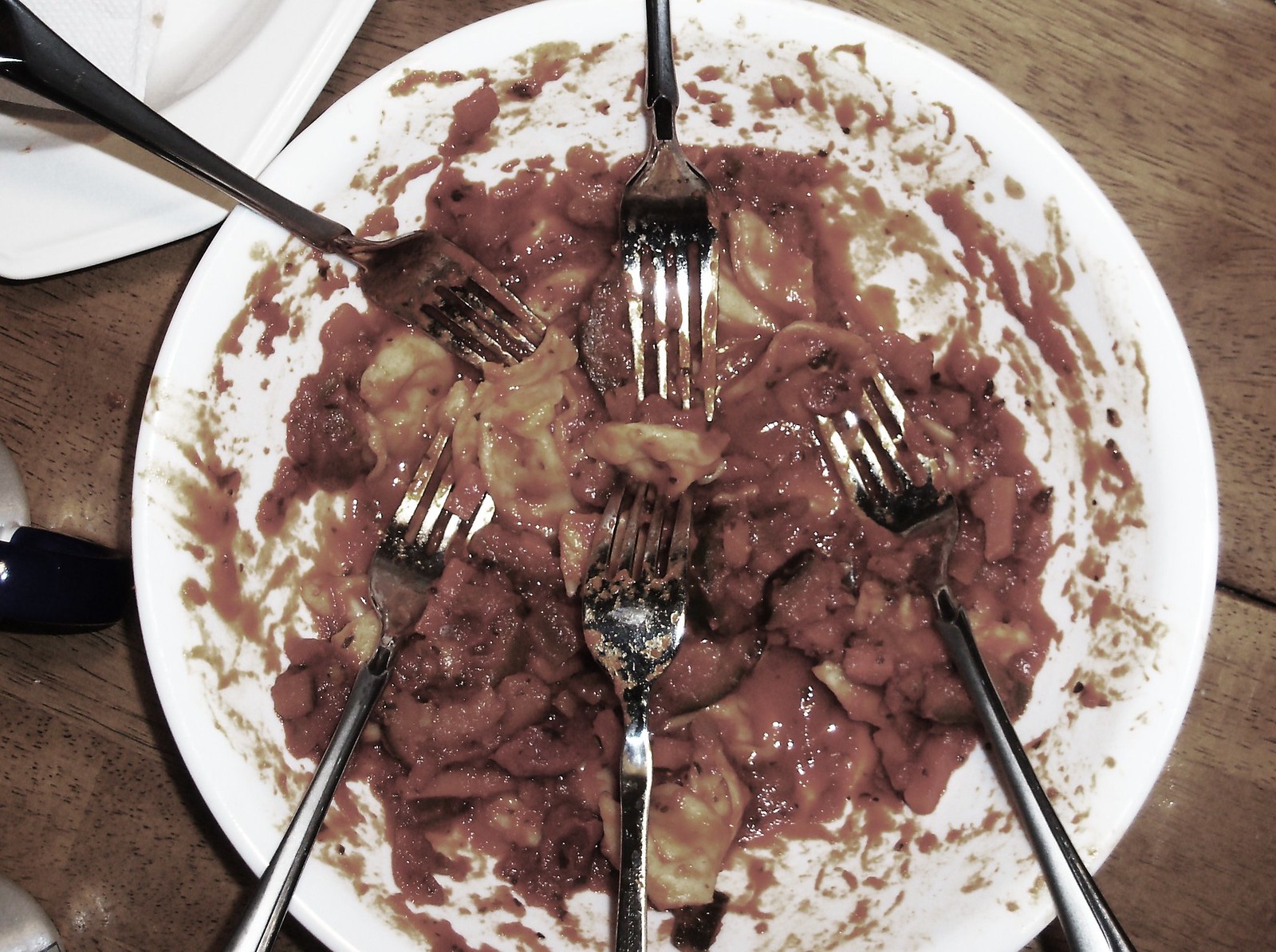The photograph displays a close-up of a tabletop scene featuring a white bowl in the upper left corner and a white plate in the middle filled with a colorful pasta dish. The wooden table, composed of a couple of wood boards, serves as the backdrop. The pasta, mixed with a rich red tomato sauce and a creamy beige to orange hue, appears messy with sauce splattered around the plate's edges. The pasta is accompanied by five silver or stainless steel forks, arranged haphazardly around the plate, with three forks pointing up and two faced down. To the left, a black object is partially visible, though its identity remains unclear. The lighting casts reflections on the silverware and the dark brown wood, adding depth and texture to the photograph.